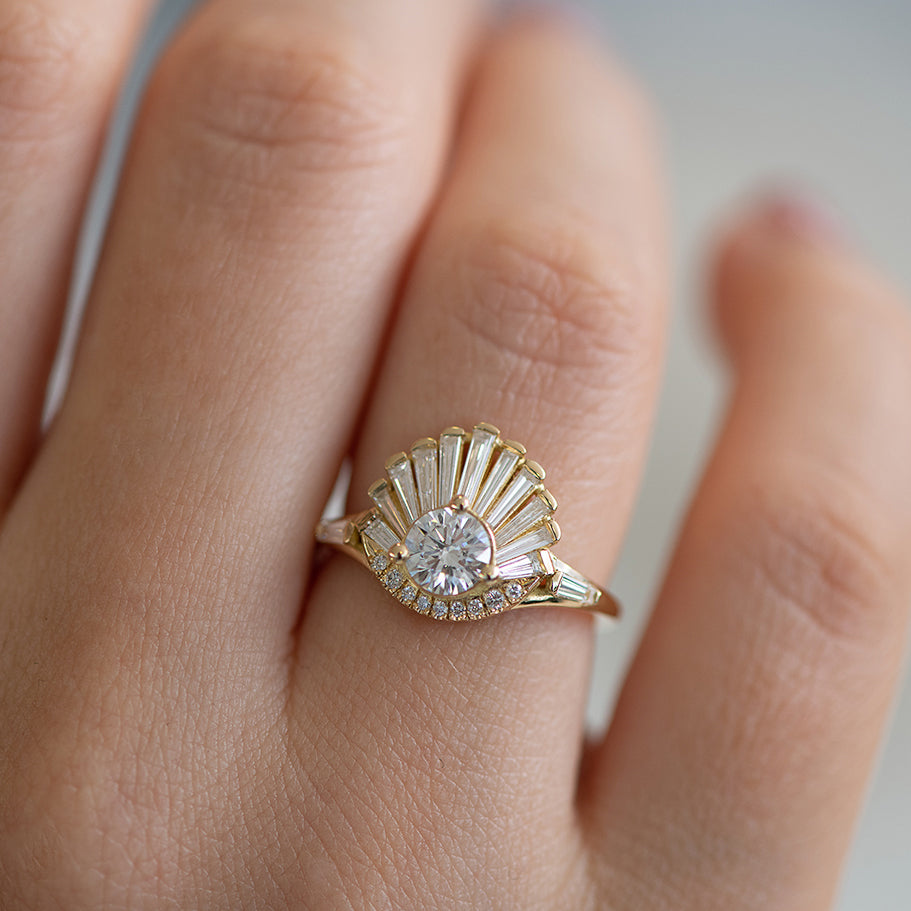This is a close-up photograph of a Caucasian female's right hand, with slightly dainty fingers adorned with light-colored nail polish on the pinky. The focus is on an ornate ring worn on the ring finger. The ring appears to be set in yellow gold and features a central round diamond, possibly a solitaire. The central diamond is flanked by a series of long rectangular diamonds that fan out in a shell-like design, resembling an Art Deco period style. Below the central diamond, there are nine smaller round diamonds set within the frame of the ring. Additional diamonds are found on the sides, highlighting the intricate and possibly expensive nature of the piece. The overall composition emphasizes the detailed and luxurious craftsmanship of the ring.